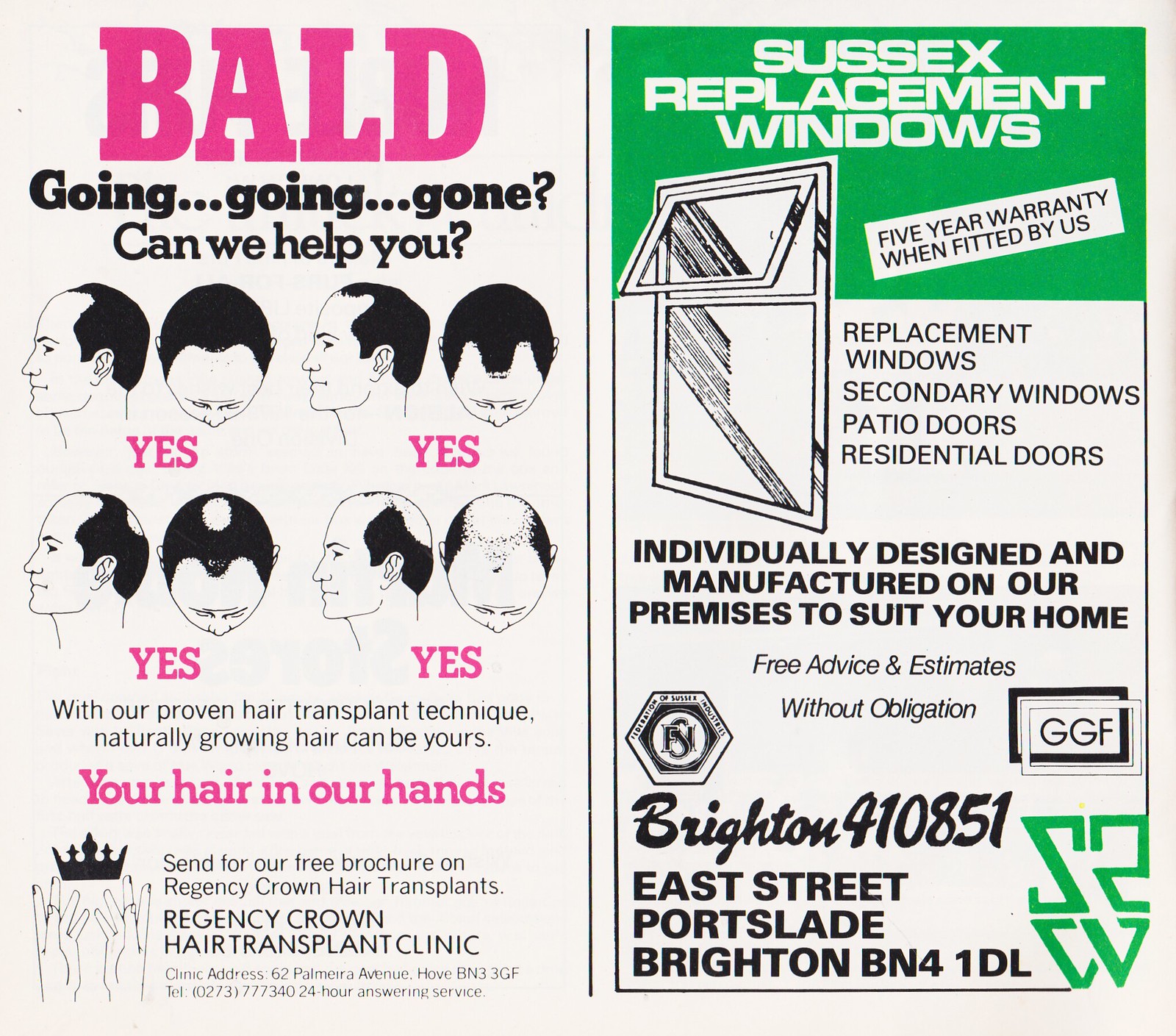The photograph captures a side-by-side display of two advertisements on a single page, likely from a magazine or similar literature. The left advertisement, set against a white background, prominently features the word "BALD" in large pink uppercase letters, followed by "GOING GOING GONE" and, "Can we help you?" in bold black font. It includes a series of four illustrations depicting a man's head at different stages of baldness, accompanied by the phrase "YES YES YES YES" in pink uppercase letters, emphasizing the capability to assist at any stage of hair loss. The text continues with, "With our proven hair transplant technique, naturally growing hair can be yours. Your hair in our hands." The advertisement further invites readers to "send for a free brochure" from Regency Crown Hair Transplant Clinic, located at 62 Palmyra Avenue, Hove BN3 3G.

On the right side, set against a green background, the second advertisement for "Sussex Replacement Windows" features a white font and an illustration of a window. It touts a five-year warranty on replacement windows, secondary windows, patio doors, and residential doors, when fitted by the company. The ad highlights the custom design and manufacturing process: "Individually designed and manufactured on our premises to suit your home." It concludes with an offer of "Free advice and estimates without obligation" and provides an address at Brighton 410851, East Street, Portslade, Brighton BN41DL.